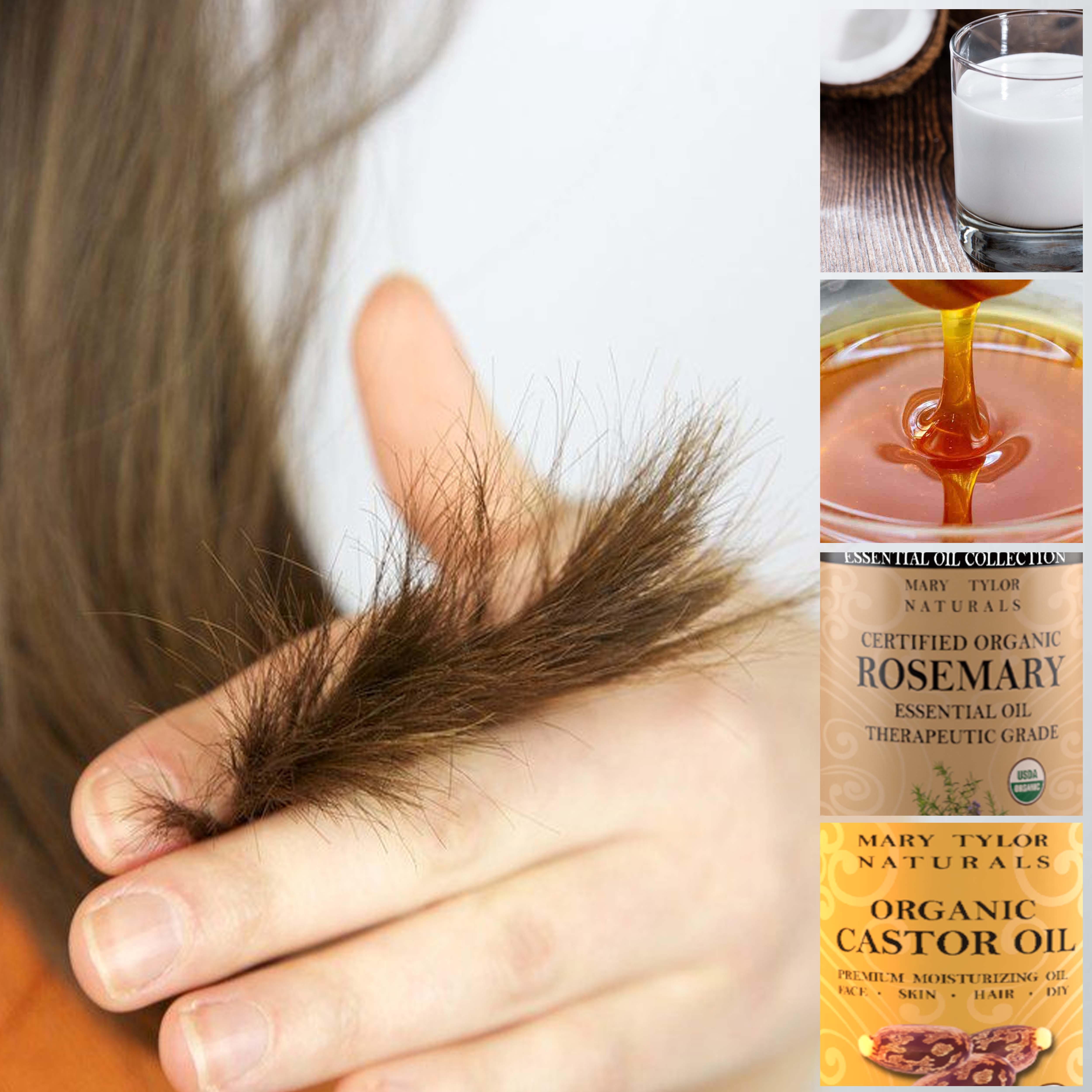This advertisement for hair care oil features a detailed composition. On the left-hand side, prominently displayed, is a close-up of a right hand with very short nails holding a chunk of long brunette hair between the index and middle fingers, highlighting the split ends against the background of an orange shirt. On the right side, the photo is divided into four smaller images stacked vertically: the top image shows a white candle in a tiny glass jar; the second depicts amber-colored honey dripping into a bowl; the third is labeled as certified organic rosemary essential oil by Mary Tyler Naturals with a brown background; and the last image features the Mary Tyler Naturals Organic Castor Oil with yellow labeling and reddish-brown bean-like graphics. This composition emphasizes the health benefits and natural ingredients of the hair care products.